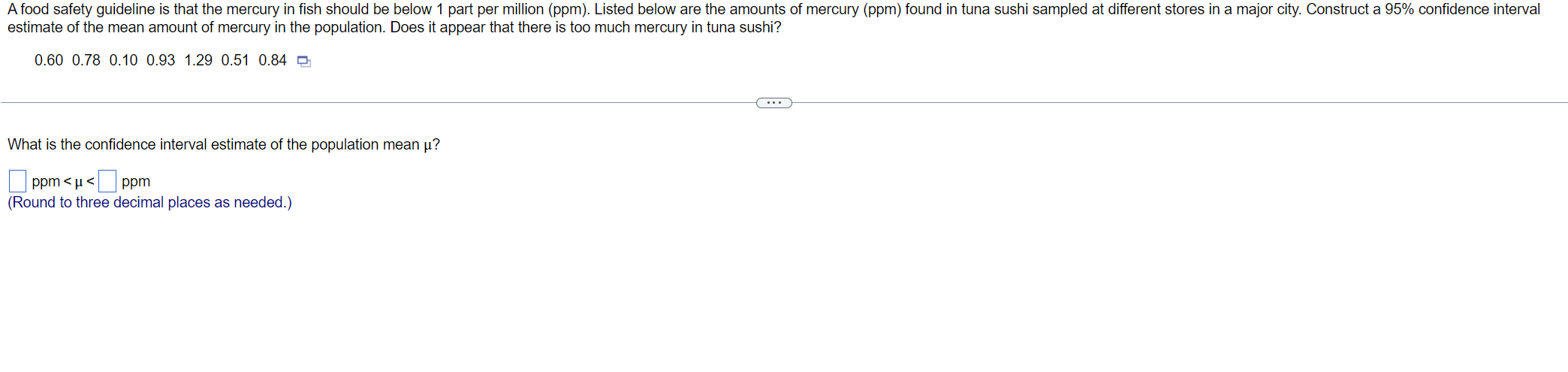The image is a screen capture from a statistics quiz question dealing with food safety guidelines related to mercury levels in fish. The top line of text, in fine black print, states that the food safety guideline requires mercury levels in fish to be below 1 part per million (PPM). It then presents a task:

"Listed below are the amounts of mercury (PPM) found in tuna sushi samples from different stores in a major city. Construct a 95% confidence interval estimate of the mean mercury level in the population. Does it appear that there is too much mercury in the tuna sushi?"

Below this instruction, a series of mercury measurements in PPM are listed:
- 0.60
- 0.78
- 0.10
- 0.93
- 1.29
- 0.50
- 0.84

Further down, another instruction asks:

"What is the confidence interval estimate of the population mean?"

Following this, there are two checkboxes with labels. The first, currently unchecked, corresponds to "PPM > μ" and the second checkbox, also unchecked, corresponds to another unknown value "PPM". The instruction "Round to three decimal places as needed" is noted in parentheses below this section.

The layout and content suggest that this image is a snapshot from a quiz or an example of a question you might see in a statistics course.